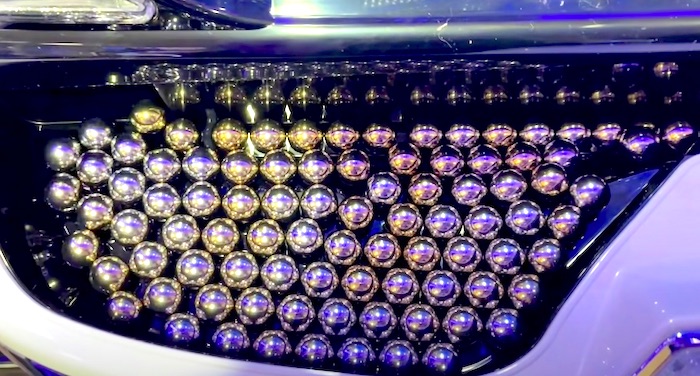This photograph presents an intriguing, abstract image of what appears to be an array of metallic, shiny spheres arranged in a meticulously organized pattern. Centered within the image, these spheres, resembling crystallized or diamond-like objects, are nestled within a sleek, reflective surface that seems to be made of porcelain. The spheres are aligned in neat rows, with around 50 of them forming a striking visual. The reflective surface beneath them appears black and glossy, with the spheres casting bright reflections upon it. A black or dark gray band runs horizontally across the top, adding to the complexity of the image by mirroring the luminous glow of the spheres, enhanced by ambient light hitting them at various angles. The overall image captures the intricate interplay of light and reflection, giving the scene a somewhat ethereal quality, with subtle hues of purplish-pink and blue adding to its abstract allure.